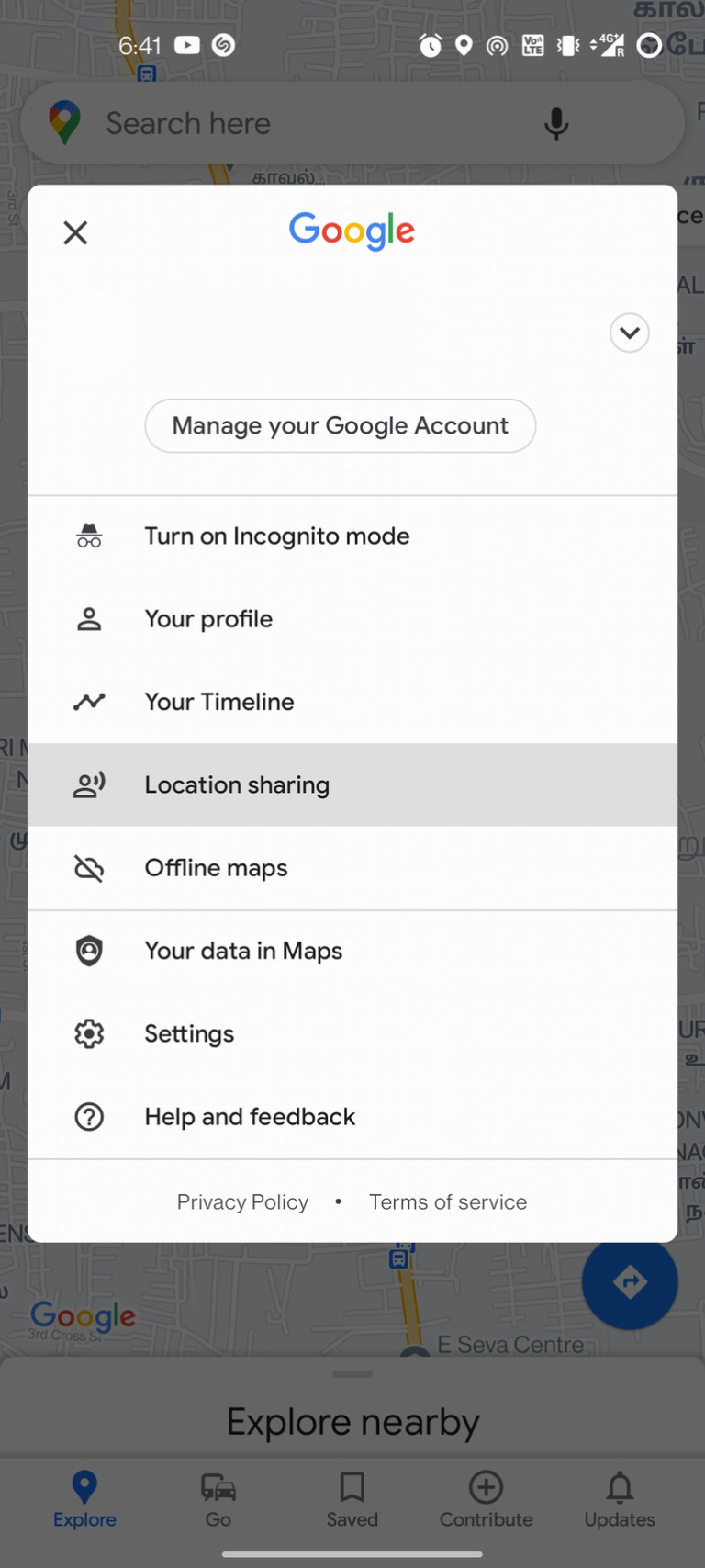This is a detailed description of a screenshot taken on a smartphone. 

In the top left corner, the current time is displayed as 6:41 AM. The top right corner features an alarm clock icon along with a location pin, and several indeterminate icons alongside these. Below this area, the background appears grayed out, creating a slightly blurred effect. 

At the center of the screen, there's a search bar containing a location pin and a microphone icon. Partially visible underneath the search bar is a portion of the Google Maps interface, displaying some roads and various locations. The words "Explore Nearby" are prominently shown, accompanied by a button labeled "Explore". Next to the "Explore" button are other buttons labeled "Go," "Save," and "Configure".

Toward the lower part of the screen, a white popup box overlays the content. In the top left corner of this box, there is a small X icon to close the popup. At the top-center of this box, the Google logo is visible in its traditional blue, yellow, green, and red colors. To the right of the Google logo, there's a dropdown menu button. 

Below this, a button labeled "Manage your Google Account" is positioned. A light gray horizontal line separates this section from the following options. Underneath the line, options are listed: "Turn on Incognito Mode" and "Your Profile."